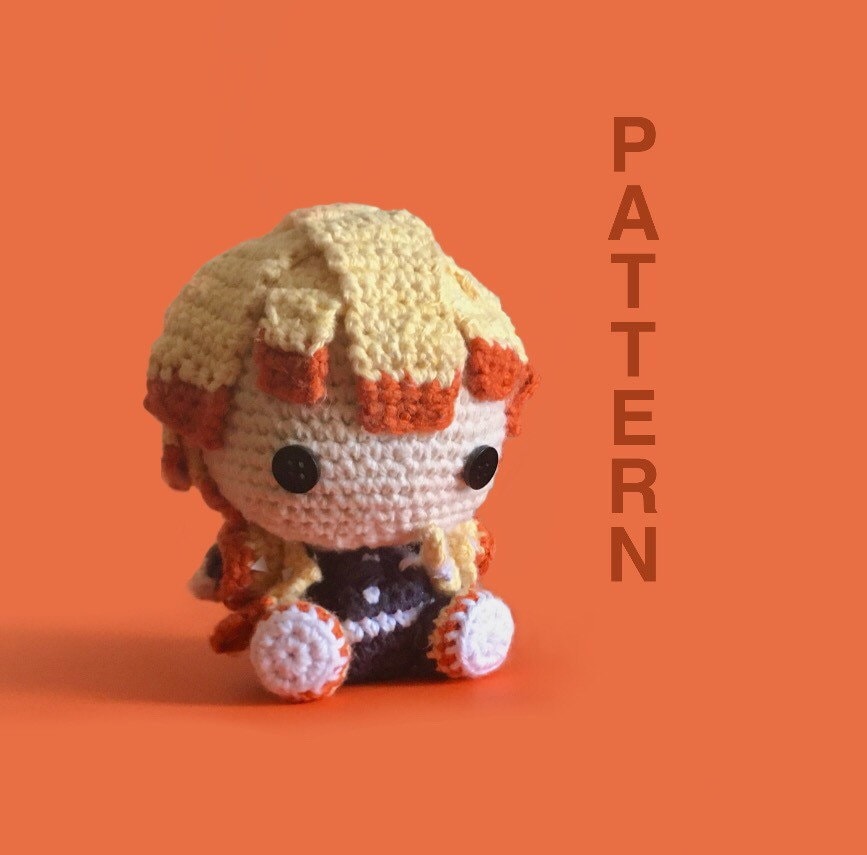In the photograph, a small crochet doll is seen against a solid, very orange background. The doll features a white crocheted face with two black button eyes and hair that is predominantly yellow with distinct red tips. It wears a black shirt and small feet that are white with an orange border. The doll is sitting on the floor, dressed in a vest that matches the color of its hair—yellow with orange accents. To the right side of the image, the word "PATTERN" is written vertically in bold, dark orange letters, standing out against the lighter orange background.